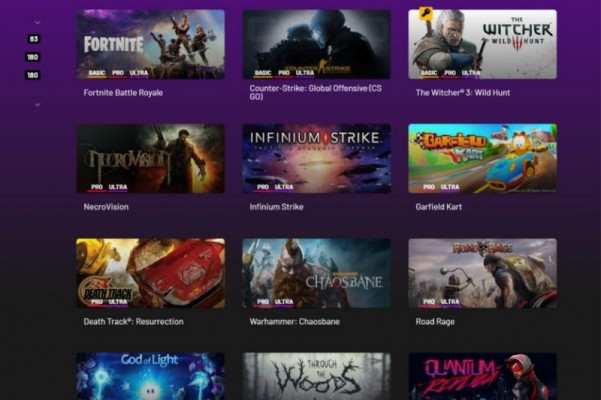The image is a vertical rectangular portrait, resembling the shape of a laptop screen. The backdrop is purple, fading to almost black near the bottom and the bottom right, giving it a gritty and gradient texture. In the center of the image, there are 12 movie or game thumbnails arranged in a grid, indicating a selection screen for choosing a movie or game to watch or play.

On the left side of the screen, there's an empty panel with a blank purple background. At the top of this panel, there are three small, dark icons with white details that are not clearly describable.

To the right of the panel, there are three full rows and a partially visible fourth row of thumbnails, each showing a full-color, landscape-oriented image representing the respective movie or game. These thumbnails are almost twice as wide as they are tall. Below each thumbnail, there is left-justified white text providing the title of the movie or game. 

The first thumbnail in the upper-left corner features an image from "Fortnite Battle Royale" which depicts three characters firing futuristic rifles. Below each thumbnail, in the lower-left corner, are three all-caps words in white: BASIC, PRO, and ULTRA. These are tier indicators, with BASIC showing a yellow line, PRO a red line, and ULTRA a purple line. Not all thumbnails have the BASIC tier; some only show PRO and ULTRA. 

The second thumbnail shows "Counter-Strike: Global Offensive (CS:GO)," featuring two soldier-like characters in a dark, futuristic setting. The far-right thumbnail in the top row is "The Witcher 3: Wild Hunt," displaying a character in medieval armor reaching for a sword.

In the second row, the thumbnails are "Necrovision," "Infinium Strike," and "Garfield Kart." The "Garfield Kart" thumbnail features a cartoonish image of Garfield in a light blue racing car. These do not have the BASIC tier, only PRO and ULTRA.

The third row showcases "Death Track Resurrection," "Warhammer: Chaosbane," and "Road Rage." The "Death Track Resurrection" thumbnail shows a red car performing a wheelie, while the "Warhammer: Chaosbane" image is very busy with detailed artwork. 

The fourth row, partially cut off, includes "God of Light," "Through the Woods," and a partially visible "Quantum" title, possibly "Quantum Rapture." The "God of Light" thumbnail is predominantly blue, "Through the Woods" has a light gray and brown motif, and the "Quantum" title shows a figure in a hood.

This selection screen likely allows users to choose from these movies or games to watch or play.